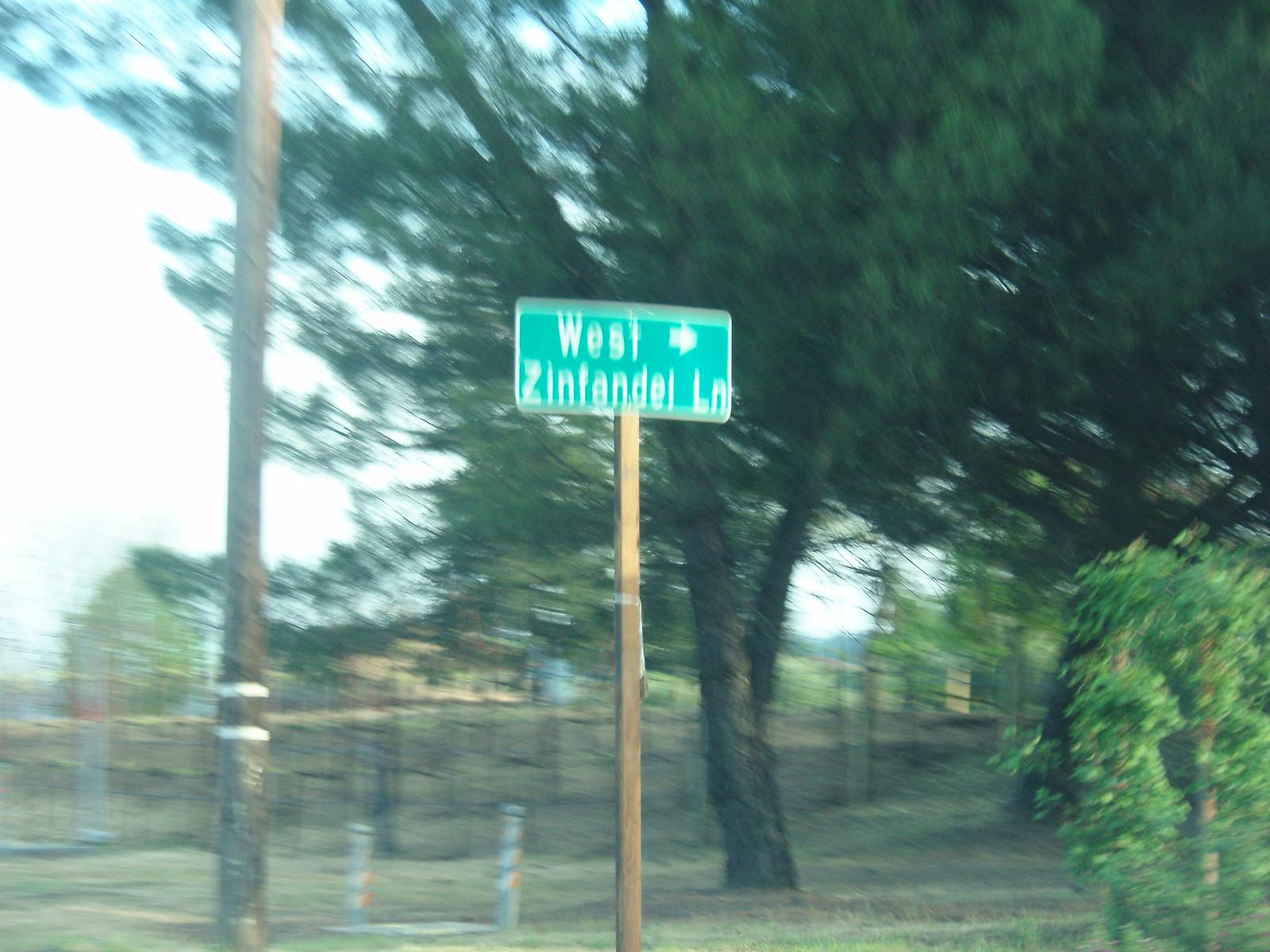A daytime photograph, slightly blurry and seemingly taken from a moving vehicle, captures an urban scene centered around a green street sign with white text reading "West Lane" and an arrow pointing to the right. Directly to the right of the sign, a bush with pale green foliage is visible, while to the left stands a brown wooden telephone pole encircled by two silver metal wires. Dominating the background is a large tree with lush, dark green leaves, accompanied by another tree partially hidden behind it. The scene appears to be situated alongside a walking path, beyond which lies a vast field. In the far background, a cream-colored building can be seen, adding to the landscape's depth.